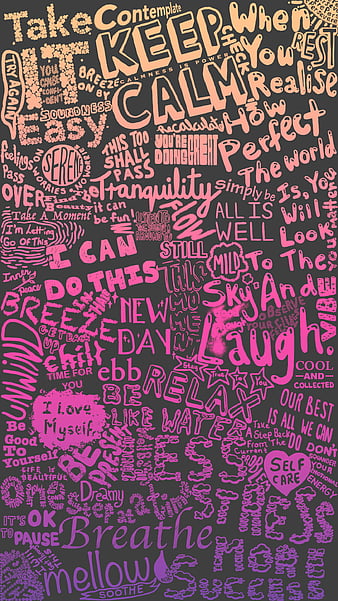The image features a black background filled with an array of uplifting words and phrases printed in various fonts. The text creates a gradient effect, starting with a light brown (or peach) at the top, transitioning to hot pink in the middle, and ending in purple at the bottom. Phrases such as “Take It Easy” near the top left, "Tranquility" in the middle, and "Relax" near the bottom stand out prominently. Notably, there is a heart graphic containing the words "Self Care" and a speech bubble saying "I love myself." Other notable texts include "I can do this" on the left and "All is well" on the right, symbolizing positivity and peace. Additional comforting phrases like "Look to the sky and laugh," "Mellow Smoothie," and "Peace" are scattered throughout. The overall theme revolves around self-care, tranquility, and mindfulness, all set against a versatile black canvas that enhances the varied and vibrant fonts.